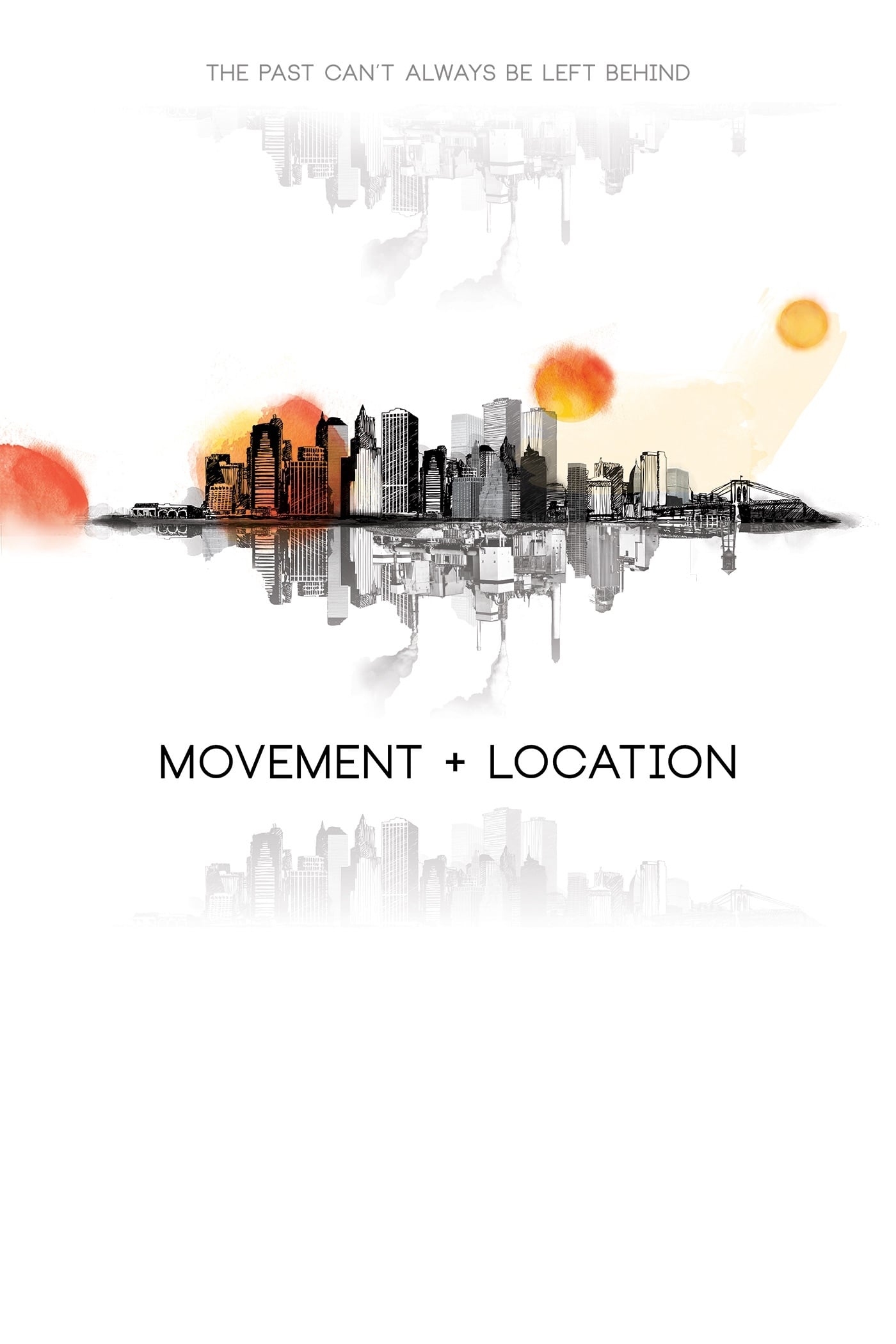The image is a detailed illustration of a cityscape presented in a square format with a central focus on a tightly packed skyline of skyscrapers, predominantly rendered in black and shades of gray. The illustration includes four distinct spherical representations of the sun, transitioning from a reddish-orange on the far left to an orangish-yellow on the far right, suggesting the passage of time or different states of the sun. These orbs add a touch of color to the otherwise monochromatic scene.

Directly beneath the city, there is a mirrored reflection of the skyline in a lighter gray, suggesting the city is set against a body of water. This reflection is accompanied by black text that reads "movement plus location." Further down, at the very bottom of the image, another lighter gray reflection of the city can be observed.

In addition to these elements, the top of the image features an inverted and grayed skyline with overlying black text stating, “the past can’t always be left behind." The cityscape is outlined against a white background, emphasizing the contrasts in the illustration. The entire composition cleverly uses spot color within a mainly black and white illustration, integrating typography to deepen the narrative of the artwork.